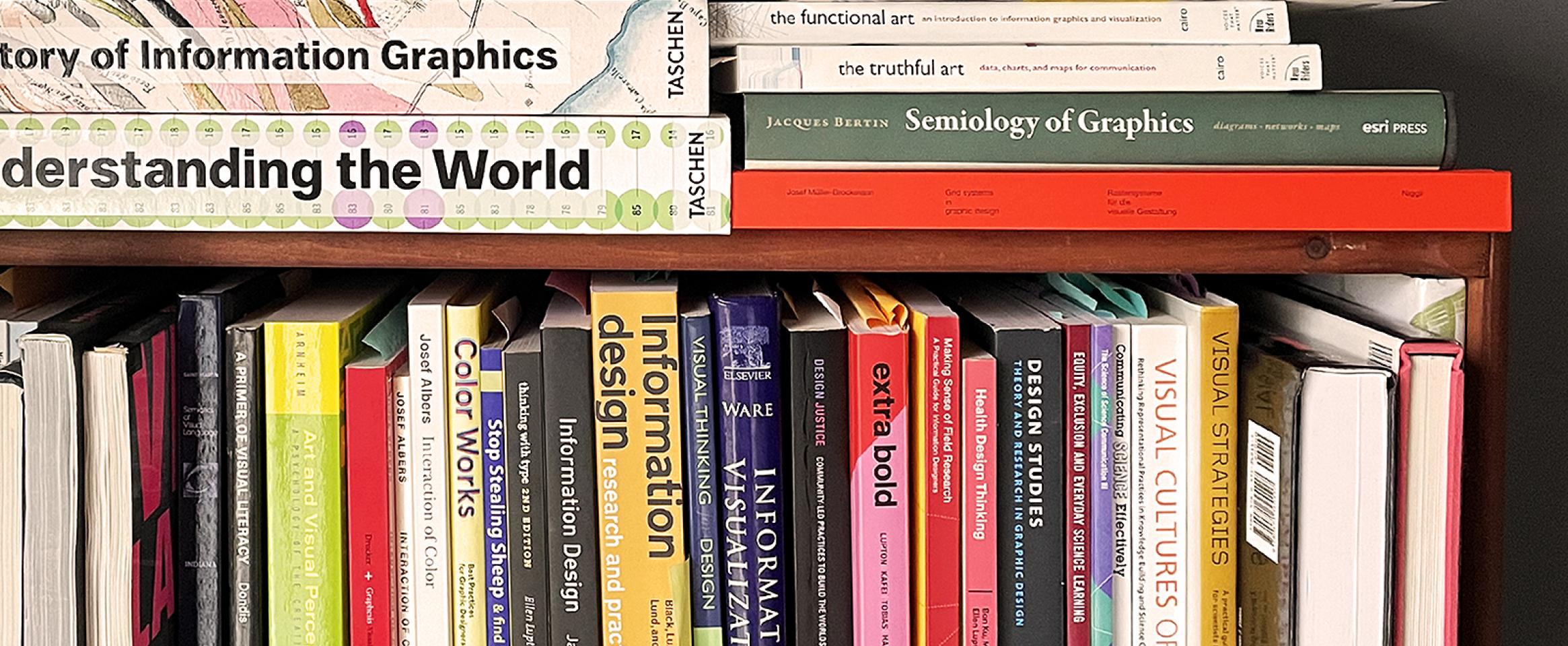The image is a full-color photograph, likely taken indoors with artificial light, depicting a meticulously arranged bookshelf. This wooden bookshelf has several rows of books, both stacked horizontally and placed vertically. The top shelf features books laid on their spines, showcasing an array of colorful book jackets. The next row down contains taller books, some standing upright and others on their sides, revealing their titles. 

Prominently visible book titles include "Understanding the World," "The Functional Art," "The Truthful Art," "Information Design," "Colorworks," "Extra Bold," "Visual Cultures," "Visual Strategies," "History of Information Graphics," and "Semiology of Graphics." These titles suggest a focus on graphic design, information design, and visual studies. The colors of the books span a spectrum, with noticeable shades of red, blue, yellow, black, white, brown, and various hues of purple and blue.

Most of the books appear to be softcovers, with the exception of a few hardcover volumes on the far right side of the shelf. This well-organized collection seems tailored for someone with a professional interest in design and visual communication.